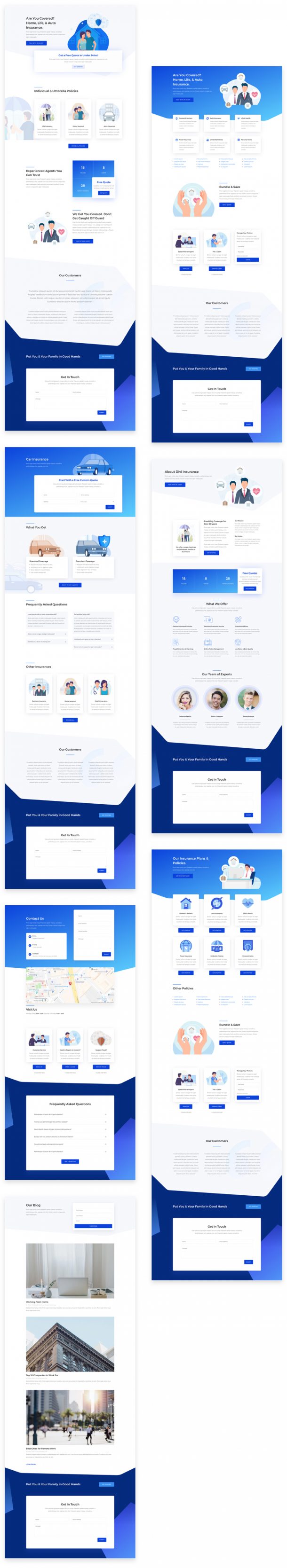This image is a screenshot displaying six distinct website templates, all presented in a compressed and miniature format, making individual elements hard to discern. The templates appear to be part of a cohesive package, given their similar layout and design elements. The arrangement consists of three templates on the left and three on the right, with those on the left being noticeably taller. 

All templates are set against a white backdrop and exhibit a general design pattern: a footer area shaded in various hues of blue, containing a white box and a hyperlink. The header sections predominantly feature a lighter blue color with embedded content, except for the first template, which has a light gray header with a picture incorporating blue tones. 

Throughout the templates, there is consistent use of text, diverse illustrations, and occasional real-life photos, enhancing the visual appeal and functional layout of each page. Each template box casts a subtle drop shadow, adding depth to the presentation. Overall, the templates incorporate different shades of blue, creating subsections and varying content fields, but the details are challenging to fully appreciate due to the image’s small and blurred nature.